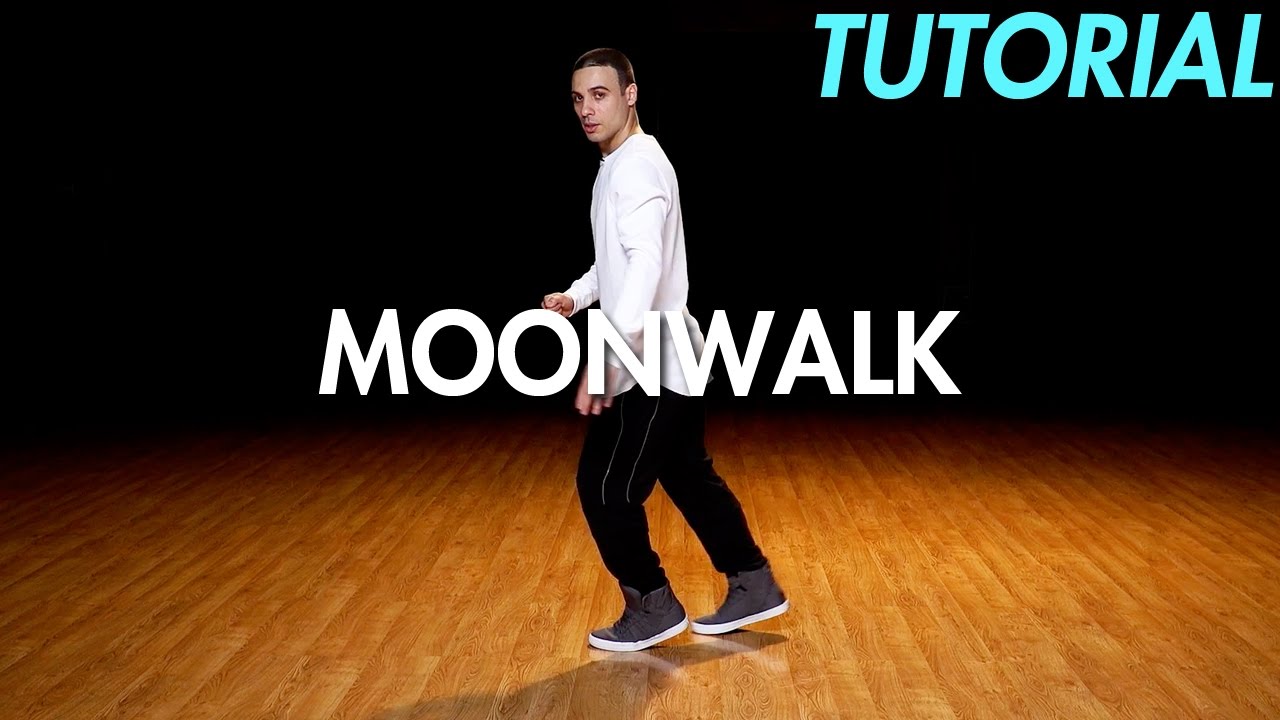The image, seemingly a screenshot from a YouTube tutorial video, features a man preparing to demonstrate the moonwalk. The man is dressed in a long-sleeved white shirt, black pants, and high-top gray sneakers with white soles. He has very short hair, possibly a crew cut, and is looking directly at the camera. He stands on a polished wooden floor indicative of a dance studio environment, while the background is entirely black, save for the spotlight centered on him. Overlaid in the image, the word "MOONWALK" appears in bold white uppercase letters across the center, and the word "TUTORIAL" is displayed in the top left corner in a bold teal color. The entire scene suggests that the man is about to teach viewers how to perform the iconic dance move.